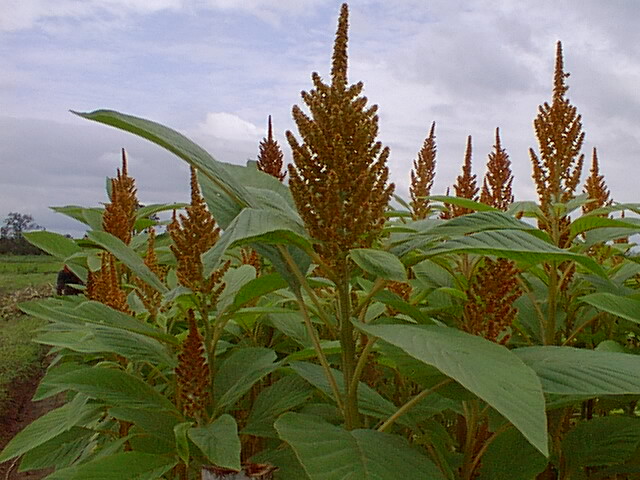The photograph features a close-up of densely clustered vegetation occupying approximately three-quarters of the frame. These plants, likely amaranth or a similar species, have large, broad green leaves shaped like ovals with pointed ends and visible ridges. The leaves are predominantly medium green, while their sturdy stems display shades of brown and yellow. Atop the stems, seed heads extend outward, bearing a fuzzy, reddish-yellow appearance, somewhat resembling pine cones.

In the background, a partially obscured human figure in a dark blue or black shirt is visible to the left, peering out from behind the plants. The lower left section of the image also reveals a strip of open, grassy field. Above the vegetation, the sky fills the upper portion of the frame, showcasing a mix of blue hues and scattered gray and white clouds. The ground beneath the plants appears to be bare earth, suggesting the scene is set in a plowed agricultural field.